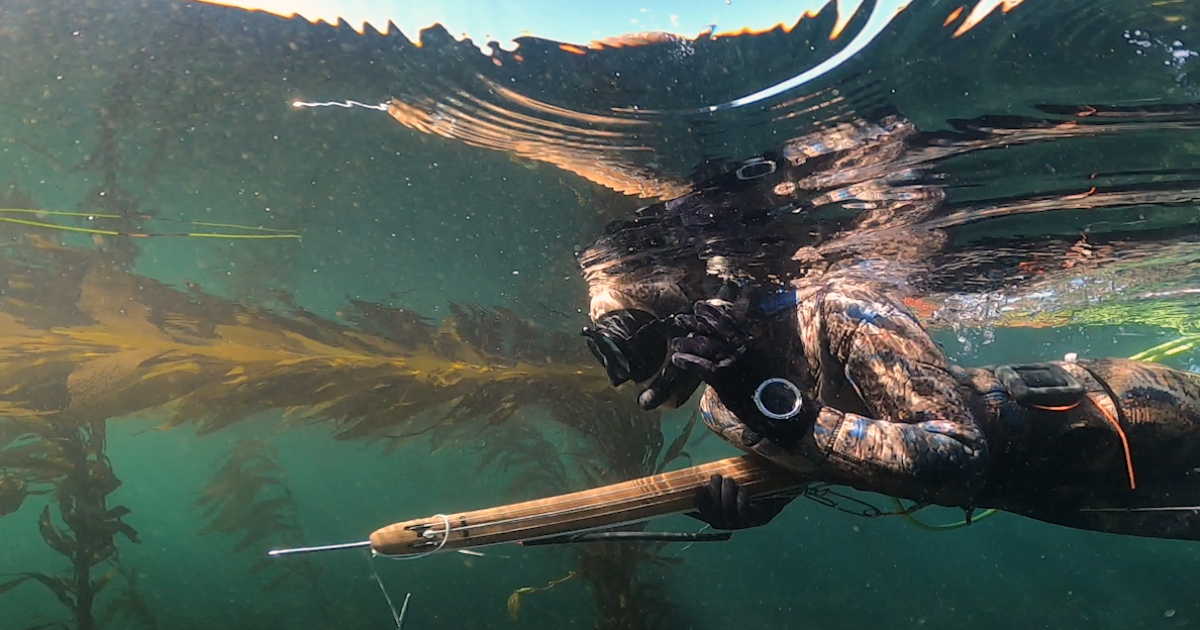The image depicts a diver swimming just below the surface of the water, illuminated by sunlight filtering down and creating vivid reflections on their upper body. The diver, potentially a woman, is dressed in a camouflage-like wetsuit with black gloves, one of which has a silver circle on it. She wears goggles, possibly a snorkel, and appears to be holding a spear gun or underwater crossbow in her right hand while her left hand is positioned near her ear. Additional equipment includes a pouch on her back and a dive watch on her wrist. She has tattoos that feature blue and black ink. The water around her is a greenish-teal color, teeming with underwater plant life, including kelp and seagrass. The scene captures the interplay of light and color, with waves and ripples visible above, adding depth to the underwater environment.